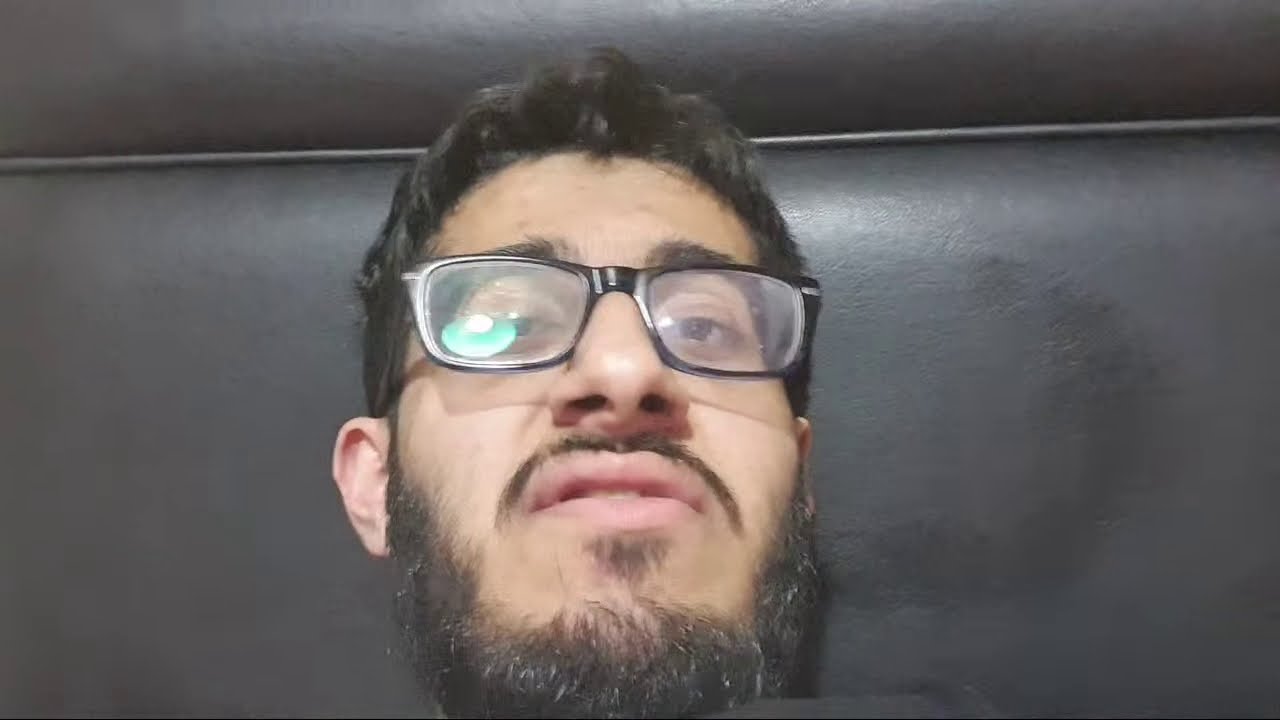This image captures a close-up view of a man, likely in his early 30s, with Middle Eastern or Indian features. He has an olive complexion, brown eyes, and short, dark hair that is covered by a tightly-knit cap. The man is wearing black, square plastic-rimmed glasses with distinct horned edges at the top corners. His facial hair includes a scraggly, slightly unkempt beard with patches of gray and a thin, less substantial mustache. The photograph appears to be taken from a lower angle, as if the camera is looking up at him, contributing to a somewhat awkward perspective.

The man's expression shows his mouth slightly open, suggesting he might be in the middle of speaking, or perhaps it's just his natural expression which comes off as a bit disdainful. He seems to be making eye contact with the camera, possibly hinting at an interaction such as an interview. Blurred in the background, a black, padded wall with visible seams and reflections from a light source in his glasses indicate an indoor setting, potentially a train or a room with black leather seating.